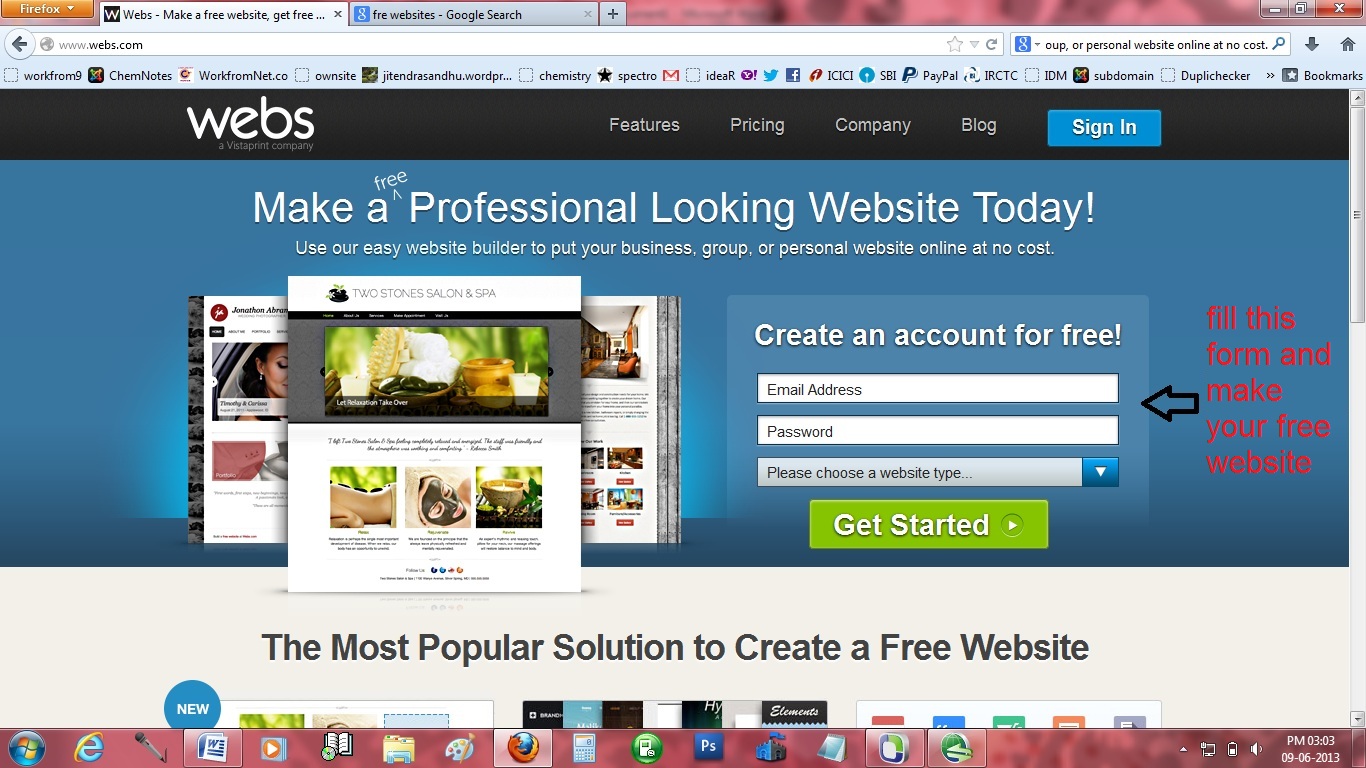This screenshot captures the homepage of the website "www.webs.com." At the very top of the page is a search bar displaying the URL. The header banner is black with the word "webs" written in lowercase white letters on the left side. On the right side of this banner, there are navigation links labeled "Features," "Pricing," "Company," "Blog," and "Sign In."

The central section features a background in hues of blue. Dominating this area is an image of a webpage for "Two Stones Salon and Spa." This primary image partially overlaps several other websites displayed behind it. Overlaying this visual, there is bold text that reads, "Make a free, professional-looking website today. Use our easy website builder to put your business, group, or personal website online at no cost."

Beneath this text, there is a call-to-action section prompting users to create an account for free. This section includes fields for "Email address," "Password," and a drop-down menu labeled "Please choose a website type." The call-to-action button, labeled "Get started," is displayed in white letters within a green rectangle.

An additional arrow has been annotated, pointing toward the "Create an account for free" area, with red text stating, "Fill this form and make your free website."

At the bottom of the page, a white banner with black lettering proudly declares, "The most popular solution to create a free website."